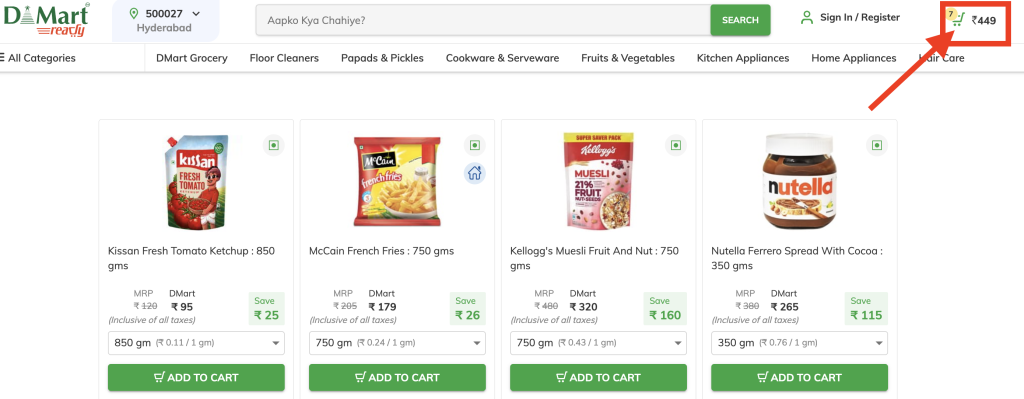A screenshot of an online shopping website featuring a clean white background. The interface is wider than it is tall. In the top left corner, a green font indicates the section, and below it, in smaller red font, is a text likely saying "Ready," although it's unclear. To the right of this section, spans the top of the page, is a drop-down menu with a number, followed by the word "HydroBad" or similar. Continuing to the right, there's a gray search bar with a green search button.

In the upper right corner, there's a sign-in/register section next to a small grocery cart icon, which is colored and outlined in red. Below the top bar, a series of category tabs span across the page, including labels such as "All Categories," "Grocery," and "Floor Cleaners," among others, totaling about six tabs.

The section beneath these tabs displays four purchasable items horizontally: "Fresh Tomato Ketchup," "French Fries," "Kellogg's Fruit and Nut," and "Nutella." Each product listing includes the price, detailed information, size, and a green "Add to Cart" button. Notably, there is a red arrow pointing from the Nutella product towards the shopping cart icon in the upper right.